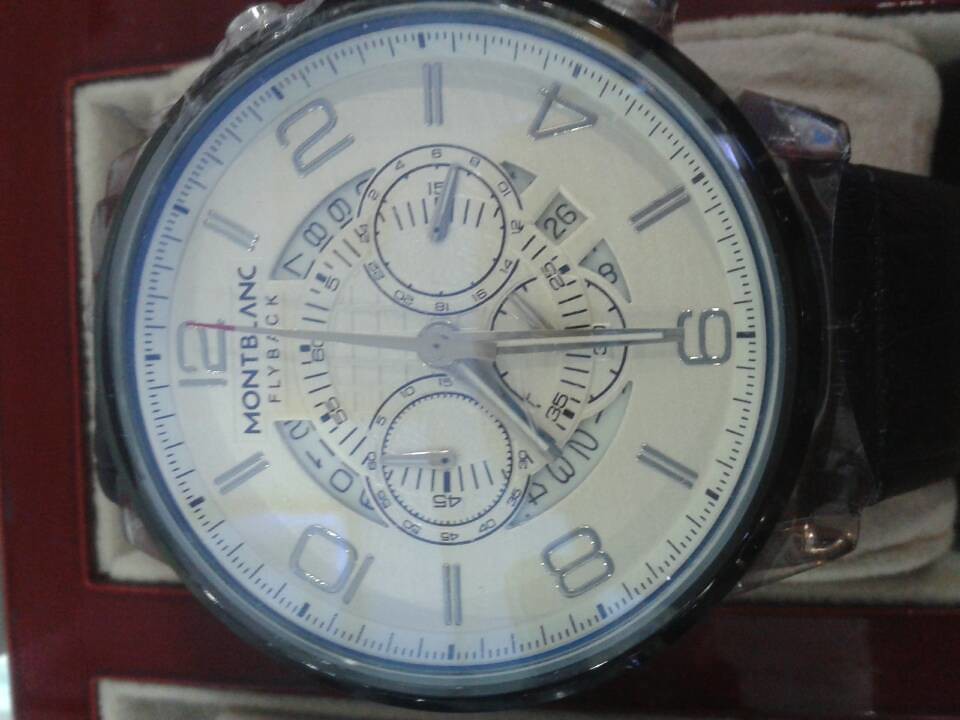A luxurious Mont Blanc Flyback watch is elegantly presented against a rich burgundy background, likely the interior of its display box. The watch rests nestled within a soft, white cushioning. Featuring a sleek black band, the timepiece is connected to its face by a polished silver piece, adding a touch of sophistication. The watch face prominently displays the brand name "Mont Blanc," although the minute or hour hand partially obscures the "L." The face design showcases only the even numbers, with two lines marking the intervals between them, and smaller numerals indicating the minutes. Centrally, the watch includes three sub-dials, each with a precise hand, providing additional functionality and detail to this exquisite accessory.